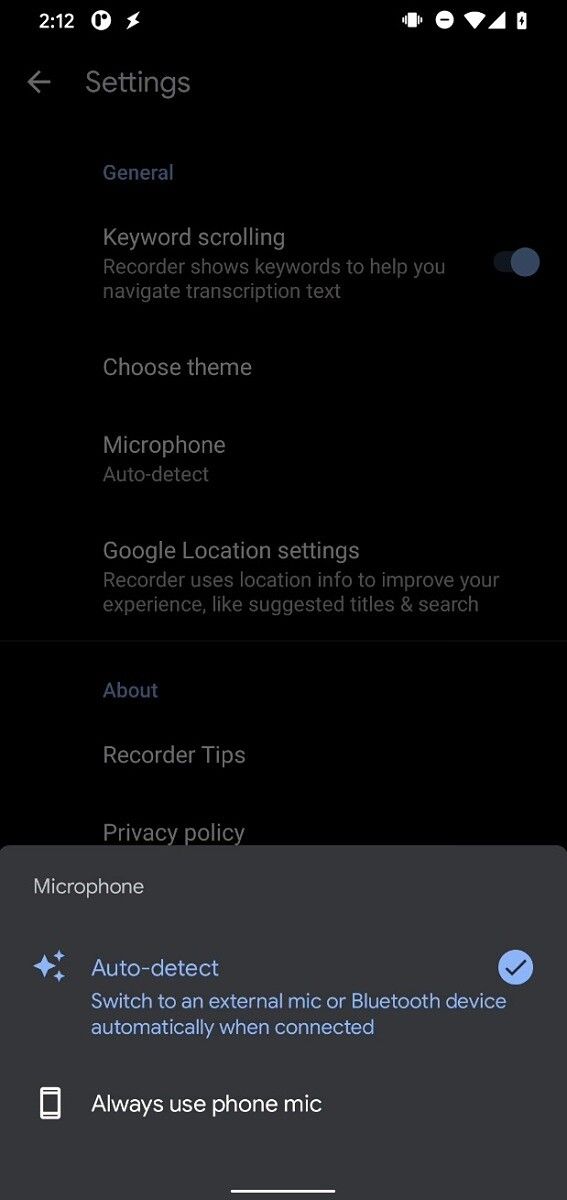The image depicts a screenshot from a mobile phone that is currently in dark mode, giving the screen a dimmed and slightly faded appearance. A gray pop-up box has appeared at the bottom of the screen, partially overlaying the interface. 

In the top-left corner of this pop-up, the word "Microphone" is displayed in white text. Below this, in blue, there are star symbols followed by the text "Auto-detect." This notification explains that if an external microphone or Bluetooth device is connected, the phone will automatically switch to it. Next to this explanation is a blue circle containing a black checkmark.

Below this section, there is an icon of a phone with the text "Always use phone mic" beside it. The entire pop-up window casts a gray filter over the rest of the screenshot.

Above the pop-up, in the top-left corner of the screen, there is a left arrow. The header displays essential phone icons, with an arrow followed by the word "Settings." Below this header are various configurable options labeled as "General," "Keyword scrolling," with an on/off toggle button, "Choose theme," "Microphone," "Auto-detect," and "Google location settings." The description under the "Google location settings" reads, "Recorder uses location info to improve your experience with suggested titles and search."